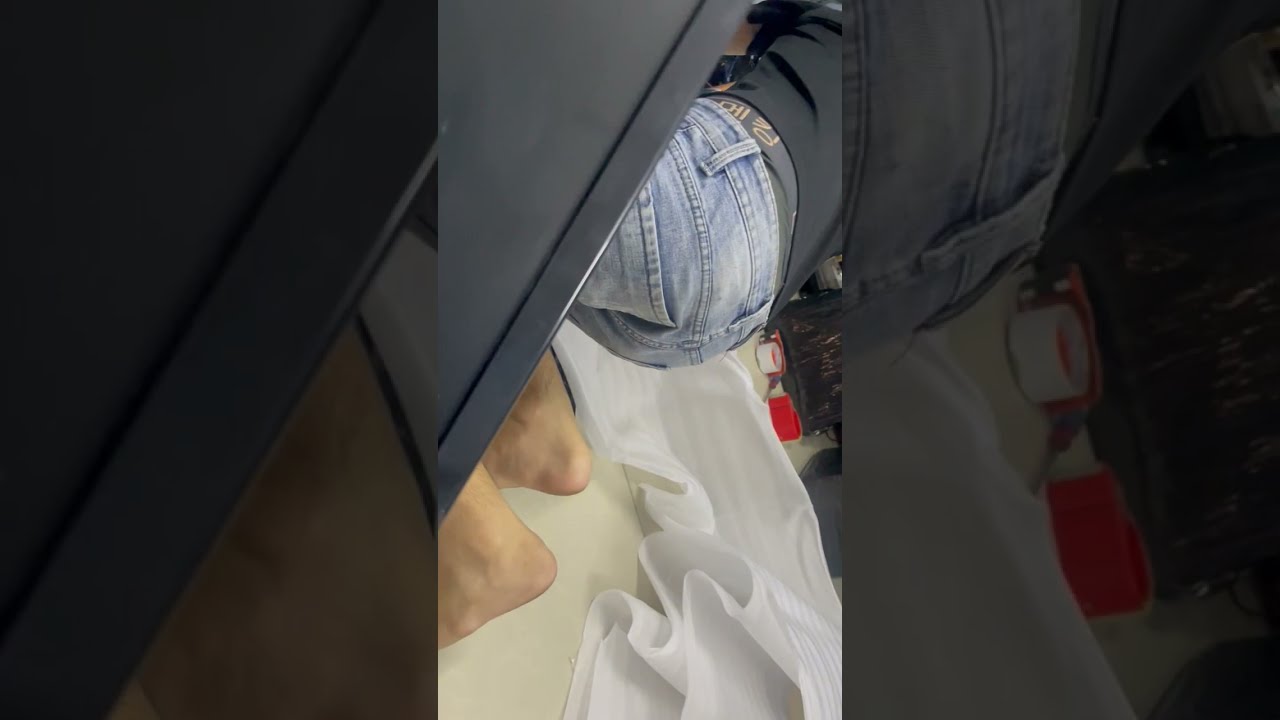In this image, there is a person, possibly a man, lying on a white sheet on the ground and working on something beneath a table. The scene is dark on both the right and left sides and is divided into three horizontal segments. From the top view, you can clearly see the individual’s feet and ankles, clothed in white footwear or socks. The person is wearing blue jeans with underwear peeking out from the waistband and a grayish shirt that is partially visible. Various items surround them on the floor, including white tape, red objects, scissors, and some black plastic covering. The overall environment suggests a scene of someone engaged in some sort of task, perhaps packing or repairing something, with a focus on their lower body and immediate workspace.